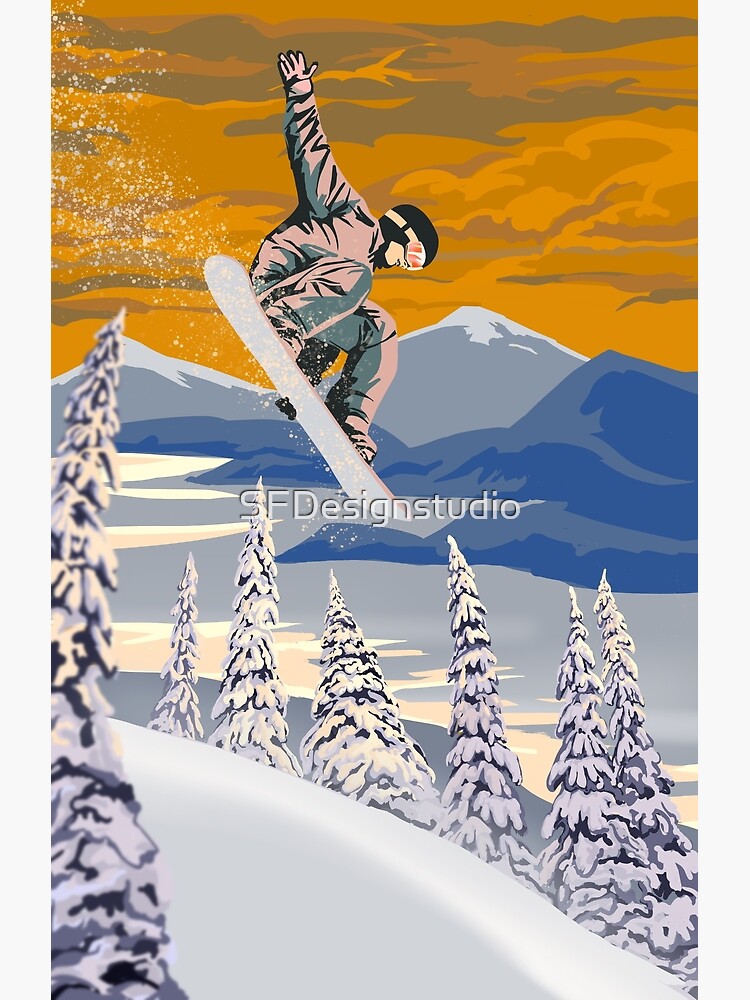This detailed 3D digital artwork captures a snowboarder mid-air against a stunning backdrop of snow-covered mountains and evergreen trees. The snowboarder, dressed in a light purple full-body snowsuit and goggles, has one hand gripping the board while the other points skyward, exuding a sense of dynamic motion and balance. His knees are bent, preparing for the descent. The snowy landscape beneath him features a gentle slope and is dotted with Christmas-like trees, particularly one prominent, slightly blurry tree in the left foreground. The scene is framed with white borders, and the sky is an unusual mustard-yellow to orangey hue, adding a unique, stylistic touch to the image.